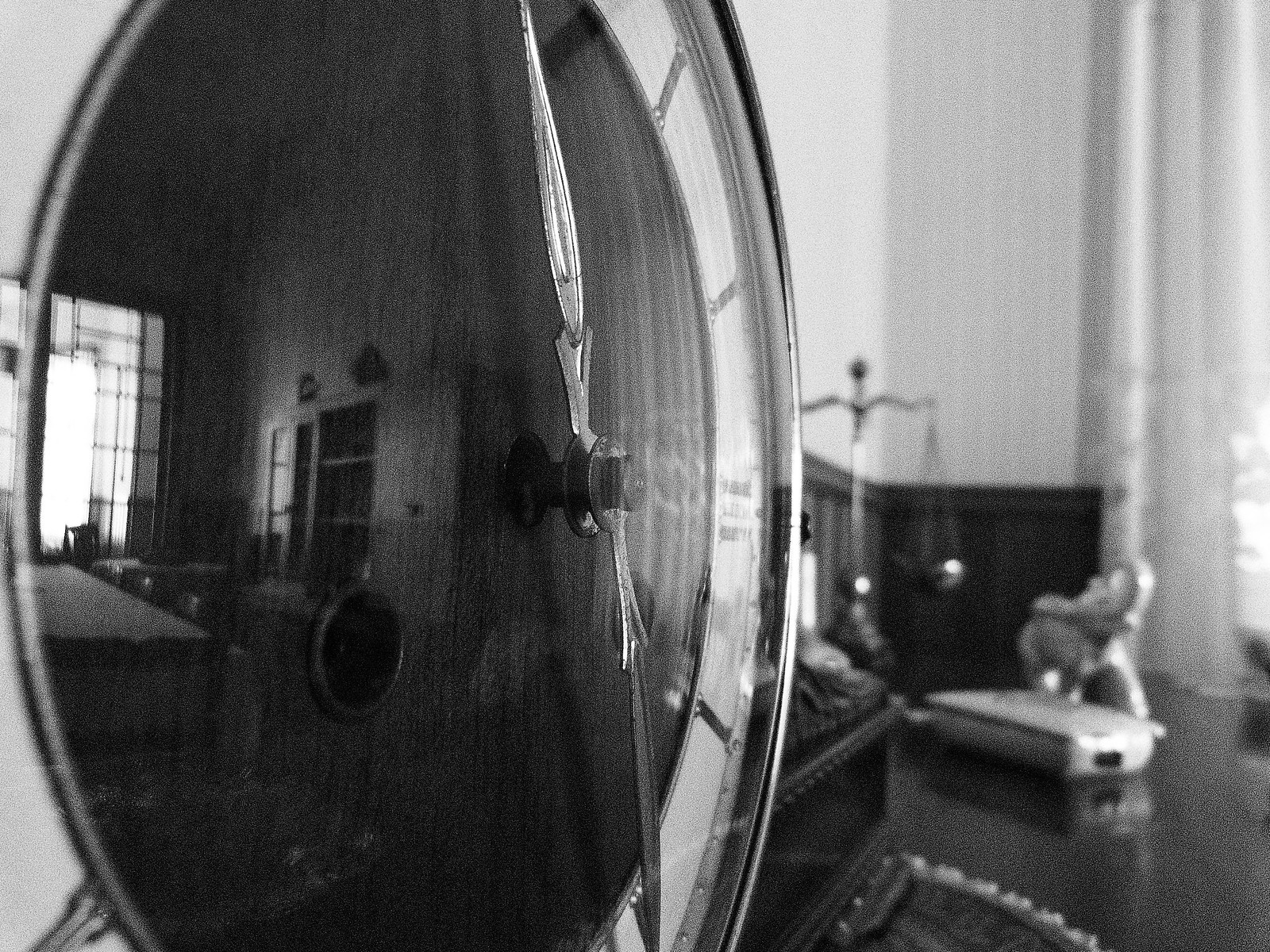This is a black-and-white photograph, artistically shot at a close-up angle of a classic clock face placed on a dark wooden desk. The majority of the clock face is polished black, creating a reflective surface that vividly captures the room behind the camera. Through the clock's reflection, elements of the room are visible, including a bed, a window, and a dresser against the wall. To the right of the image, adjacent to the clock, the desk is partially visible, adorned with an elephant statue figurine and an old-fashioned hanging balance scale, composed of a bar suspended by another bar with two weights or scale trays. The intricate interplay of reflections and shadows in this photograph adds a layer of depth and narrative to the composition.